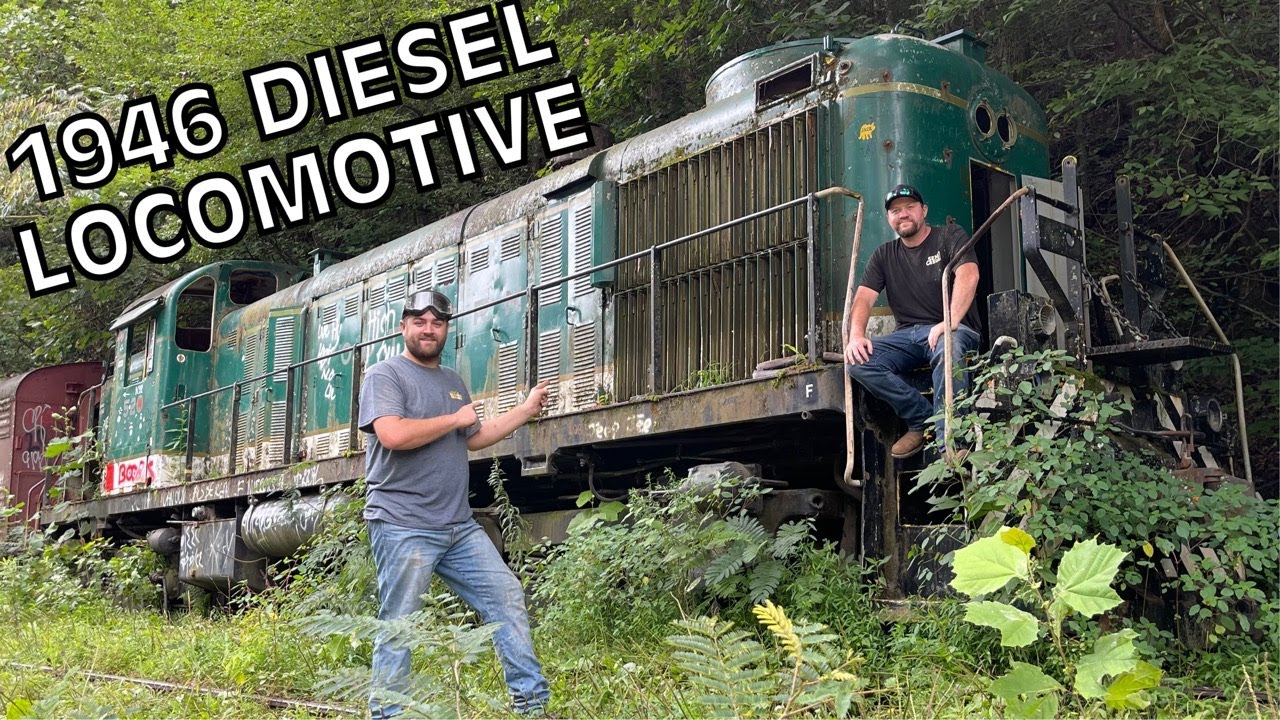In this evocative outdoor photograph, two men are seen exploring a weathered 1946 diesel locomotive, prominently labeled with white lettering in the upper left corner. The green-painted metal of the train car is heavily faded and bears marks of graffiti, evoking a sense of abandonment. The scene is set on an overgrown track, partially obscured by brush, leaves, and encroaching trees, enhancing the impression of an untamed, forested setting. The locomotive, a grayish-green color, is centrally framed, with one man sitting near its door on a small step featuring a railing. He wears a black shirt, blue jeans, black hat, and boots. The other man, standing in front of the train, points at it with a sense of discovery. He sports a gray t-shirt, blue jeans, and goggles perched atop his head. The overall ambiance of the photograph suggests a nostalgic adventure, with the two men seemingly enjoying their find amidst the wild, natural surroundings.